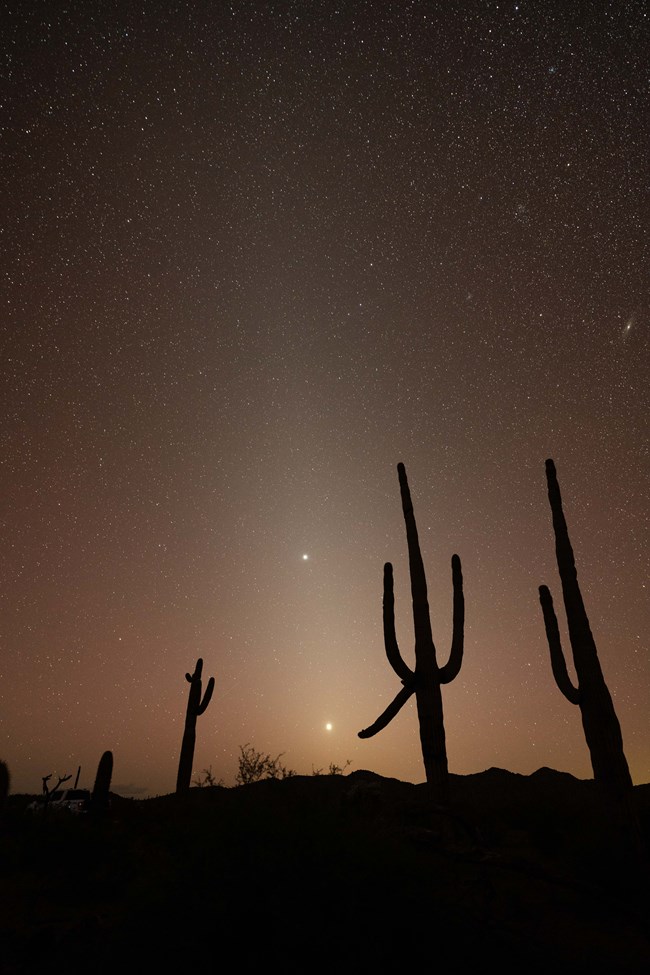The photograph captures a serene nighttime scene set in a desert landscape. The night sky, a gradient that transitions from dark purple at the top to a lighter purplish-pink near the horizon, is sprinkled with numerous stars. Two prominent points of light stand out near the middle of the sky, shining brighter than the rest, potentially stars or celestial objects. The lower portion of the image reveals the desert ground, featuring several cacti silhouetted against the varied tones of the sky. On the far right, a tall cactus with a distinctive U-shaped formation stands prominently, while to its left, several other cacti of varying shapes and sizes add to the quintessential desert atmosphere. Tumbleweeds are scattered on the ground, and what looks like a distant fence or perhaps a car in the bottom left corner adds an element of mystery to the scene. The merging of the sky's colors with the faint illumination of the horizon adds a tranquil yet enigmatic quality to this striking desert nightscape.